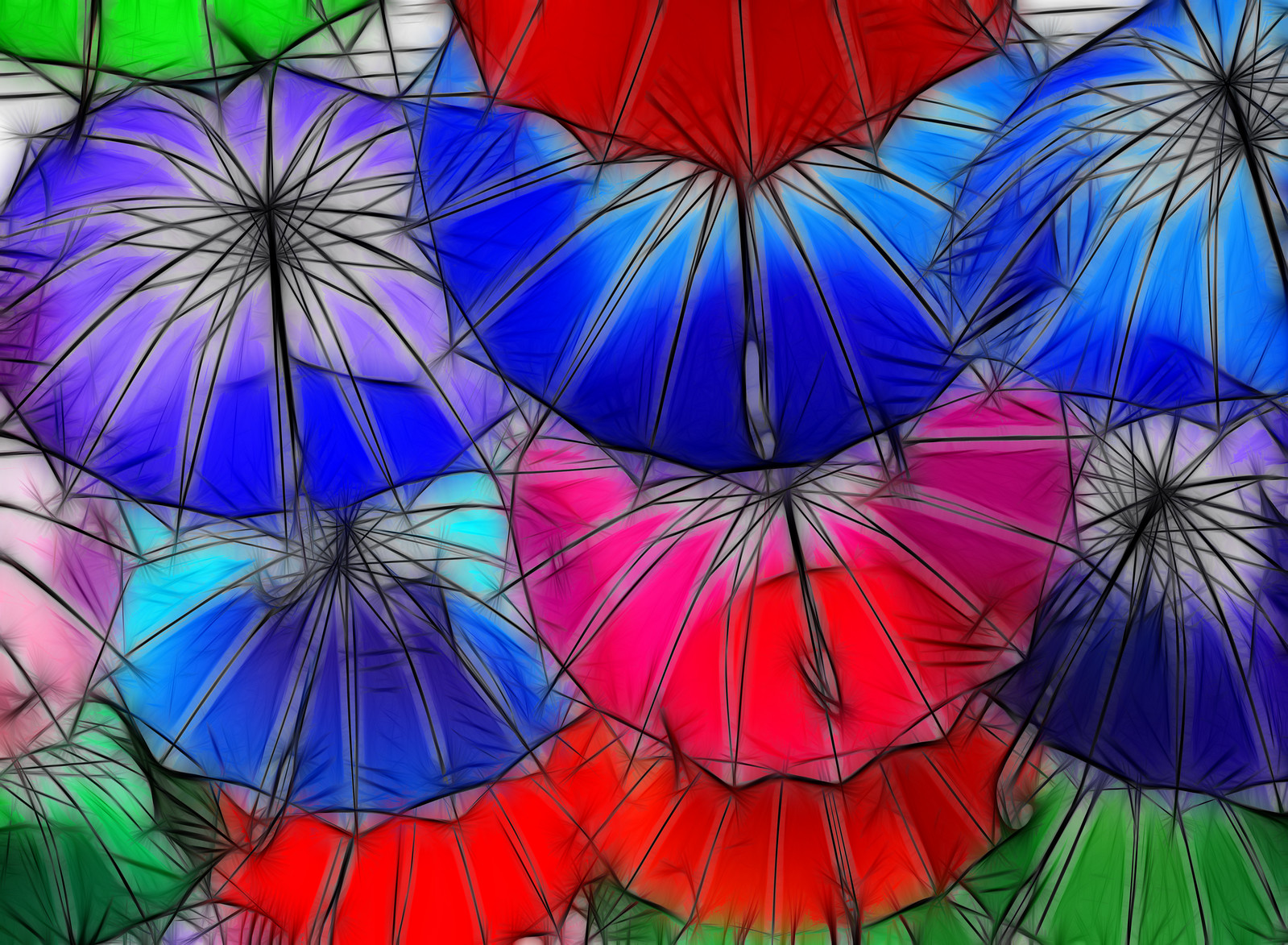This image is a vibrant digital painting of numerous overlapping umbrellas, creating a visually captivating and colorful composition. The umbrellas are arranged in an overlapping pattern that covers the entire canvas, giving the impression of a dense bouquet, reminiscent of a cluster of hydrangeas. The dominant colors include green, red, blue, purple, pink, and variations thereof, with some umbrellas appearing almost translucent where they intersect, blending their hues subtly. The artistry focuses on the dome shapes of the umbrellas adorned with black lines, giving a dynamic and somewhat sketchy impression. The handles are minimally visible, emphasizing the umbrella tops instead. The entire scene creates a playful and vivid collage that resembles a lively and dense patchwork of colorful umbrellas.